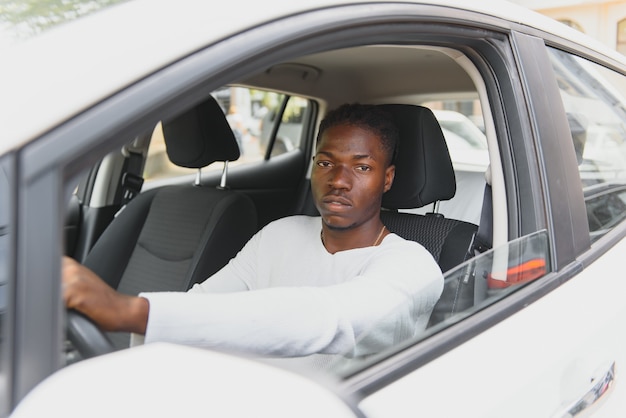In this detailed close-up photo, a young black man is seen seated in the driver's seat of a white car with clear, untinted windows. The man is wearing a long sleeve white shirt and appears to have a gold necklace chain around his neck. He has short black hair, black eyebrows, and the beginnings of a black goatee and mustache. His left hand is placed on the steering wheel, while his right hand is out of view, possibly near the gear shift. The front two seats of the car are black, with the back seats draped in white cloth. The driver's side window is rolled down, and there is a visible reddish-orange rope wrapped around a bar near the window. The door handle on the outside is silver. The man is looking directly at the camera with a neutral expression, focused on driving amid city traffic, evident by a car seen behind him. The photograph captures his moment of surprise, seemingly unsure why he's being photographed but maintaining his focus on driving.